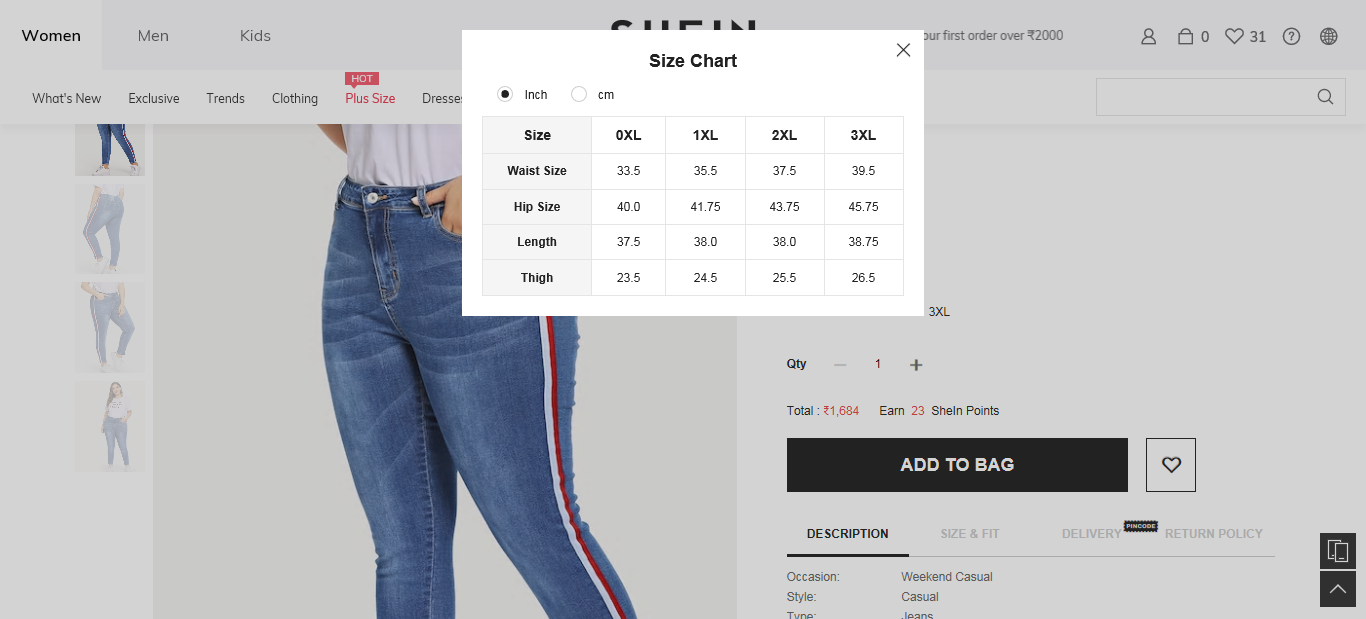Screenshot of an e-commerce website, likely belonging to the clothing retailer SHEIN, displaying a pair of jeans obscured by a pop-up size chart. The chart offers measurements in both inches and centimeters and includes categories such as size, waist size, hip size, and length. The fifth category is unclear but possibly refers to weight. The pop-up obstructs the view of the product name, making it difficult to discern the exact item being displayed. Before purchasing, users are encouraged to consult the size chart to ensure a proper fit and avoid the hassle of returns.